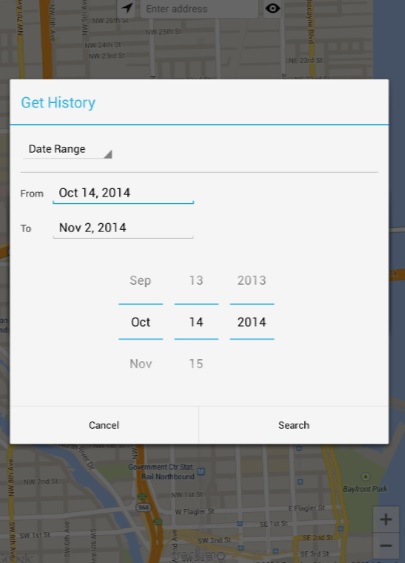A detailed screenshot of a mapping application, resembling Google Maps, depicts a gray-tinted map background obscured by a prominent white pop-up window. 

The pop-up window features the heading "Get History" in bold turquoise font at the top left corner, accentuated by a horizontal turquoise line stretching across the window. Just below the header, there is a bolded black label "Date Range" accompanied by a dropdown box.

Directly underneath, a thin light gray line spans the window horizontally. The left side of the window features the label "From," followed by the date "October 14, 2014," both in bolded black and underlined in blue. Below it, the label "To" precedes the date "November 2, 2014," similarly bolded in black, set on a gray line. 

In the center-bottom portion of the window, the date "September 13, 2013," appears in grayed-out letters with a blue underline beneath each character. However, the focus is on "October 14, 2014," which is selected and displayed in bolded black centrally with a blue underline beneath it, and the text "November 15" in gray below it.

The lower left corner of the pop-up window contains a gray-outlined rectangular button labeled "Cancel" in black, while the lower right corner features a similarly styled rectangular button labeled "Search."